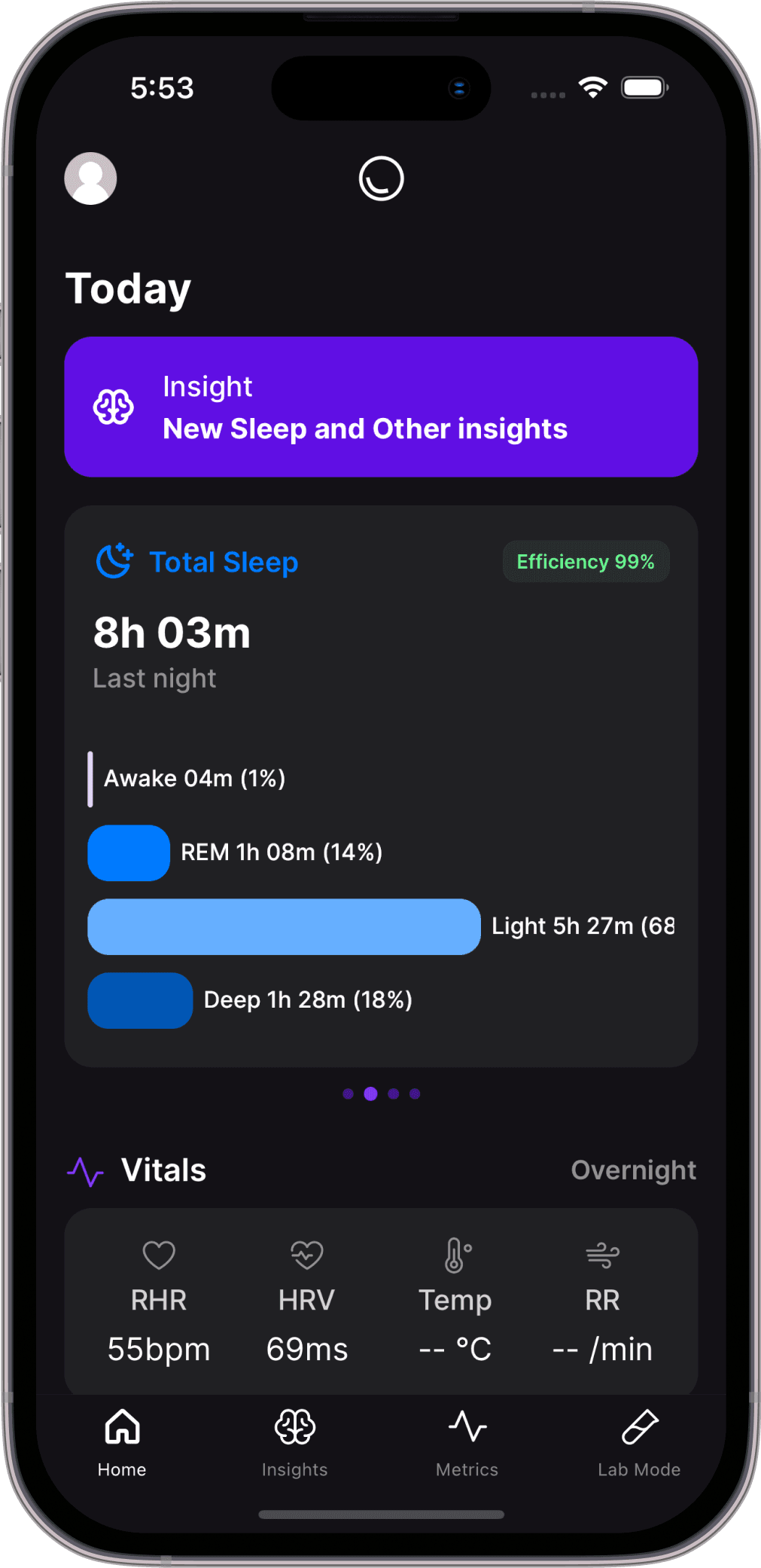This image shows a screenshot of a health or fitness tracking app, framed to appear as if displayed on a smartphone. 

The simulated phone has a grey border, highlighting the app interface within. At the very top of the screen, against a white background, the time reads 5:53 in white text. Adjacent to this is a black oval, resembling a camera placement, with a full WiFi signal icon and a fully charged battery icon in white on the right.

Beneath this header, a blank avatar icon and a small white camera symbol are displayed, possibly for profile customization. To the left, the word "TODAY" is prominently written in white. Below, a purple rectangular box with rounded corners contains white text: "INSIGHT," "NEW SLEEP," and "OTHER INSIGHTS," accompanied by a logo that is not clearly visible.

Further down, the interface features multiple elements. A grey square with rounded edges holds a moon and stars icon, labeled "TOTAL SLEEP" in blue. Below this, green text indicates "EFFICIENCY 99%," and white text logs "8 hours and 3 minutes last night." Adjacent to this, black and grey squares hint at additional interactive options, featuring blue bars likely representing sleep stages or related data.

At the bottom of the screen, there is a graph icon labeled "VITALS," displaying various health metrics, reinforcing the app’s focus on health and fitness tracking.